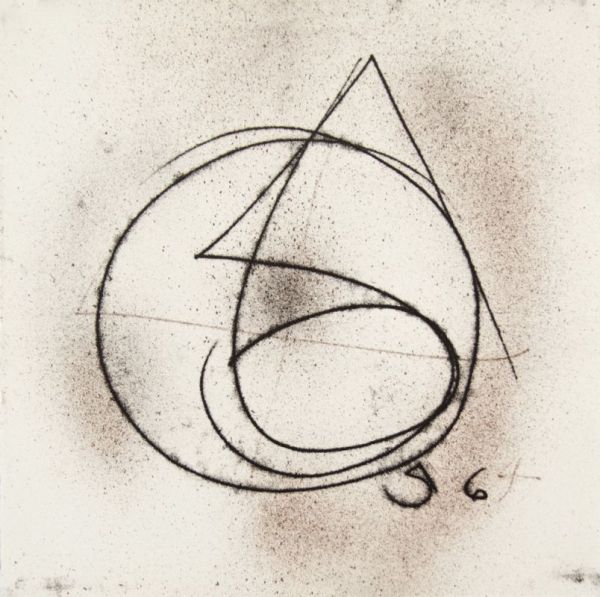The image is an abstract sketch set against a tannish white background with numerous irony red splashes scattered throughout. The entire background is splotchy and speckled with blacks and grays, evoking a sense of dirt or dust, possibly resembling a dingy piece of paper or an outdoor concrete wall.

At the center, a thin black ink circle, irregular and splotchy, draws immediate attention. Intersecting this circle is a triangular shape that culminates in a small circle at its bottom, creating a complex form. The space within the circle also includes a sketchy cross, possibly in a light brown hue.

Additionally, there are fainter black shapes, including something resembling a slanted number five and six, situated at the bottom right of the circle's outer edge. More numbers—another five and a potential faint four—are hinted at around this area. Completing the image is a prominent black splotch in the lower right corner, adding to its raw, unrefined aesthetic.